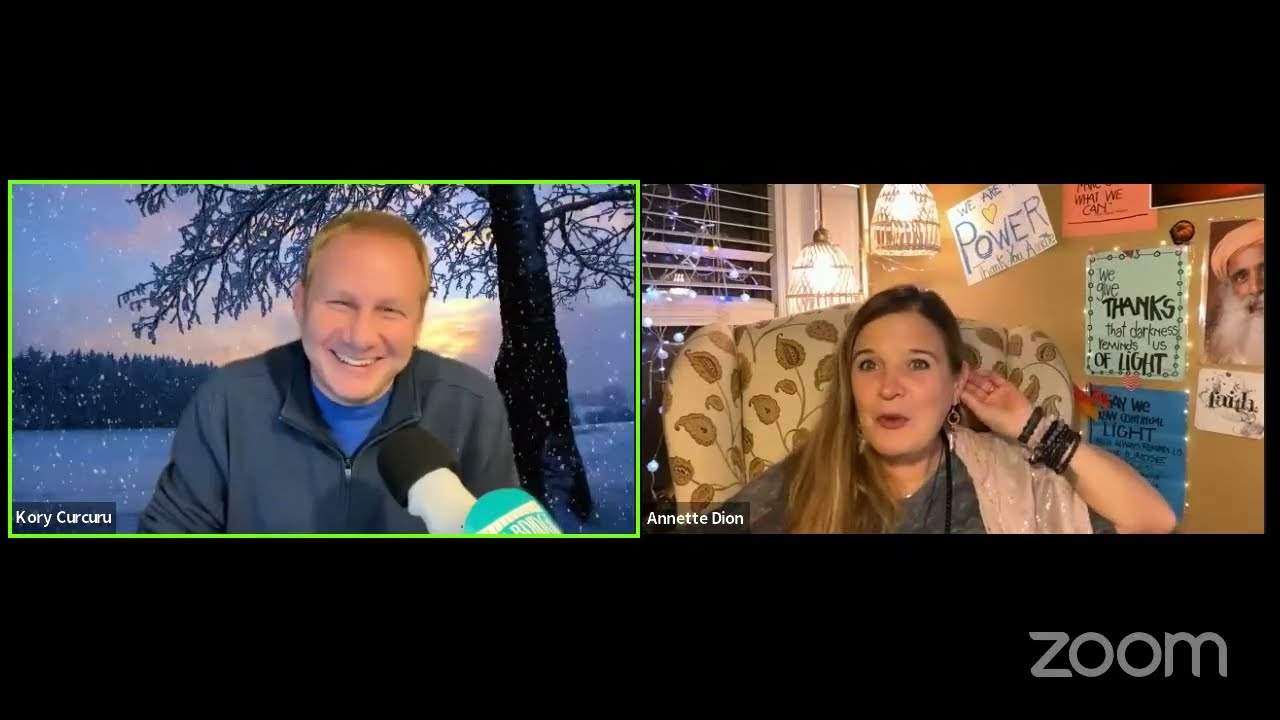This image is a detailed screen capture of an ongoing Zoom call, characterized by a black border at the top and bottom, with a gray "Zoom" watermark in the lower-right corner. The screen is split into two rectangular sections: on the left is a man, Corey Curcuru, and on the right is a woman, Annette Dion.

Corey, outlined in green indicating he is currently speaking, has short brown hair and is smiling. He is wearing a blue t-shirt under a gray quarter-zip sweater and possibly gloves, while holding a microphone. His chosen virtual background is a picturesque winter landscape featuring a tree directly behind him, a clearing with snow falling, and a tree-lined hill in the distance.

Annette Dion is sitting in a chair adorned with a floral or leaf pattern. She has long brown hair and accessorizes with multiple bracelets on her left wrist. She is wearing a gray blouse, and her environment includes a mix of bohemian elements such as hand-drawn signs, pictures, and possibly rustic or bohemian lights. Behind her, a window with vertical blinds reveals a nighttime sky, suggesting it is evening. On the wall behind Annette are hand-drawn signs, one of which reads "We Are Power," along with other child-like drawings and a picture of Santa Claus, adding a touch of personal and festive decor to the scene.